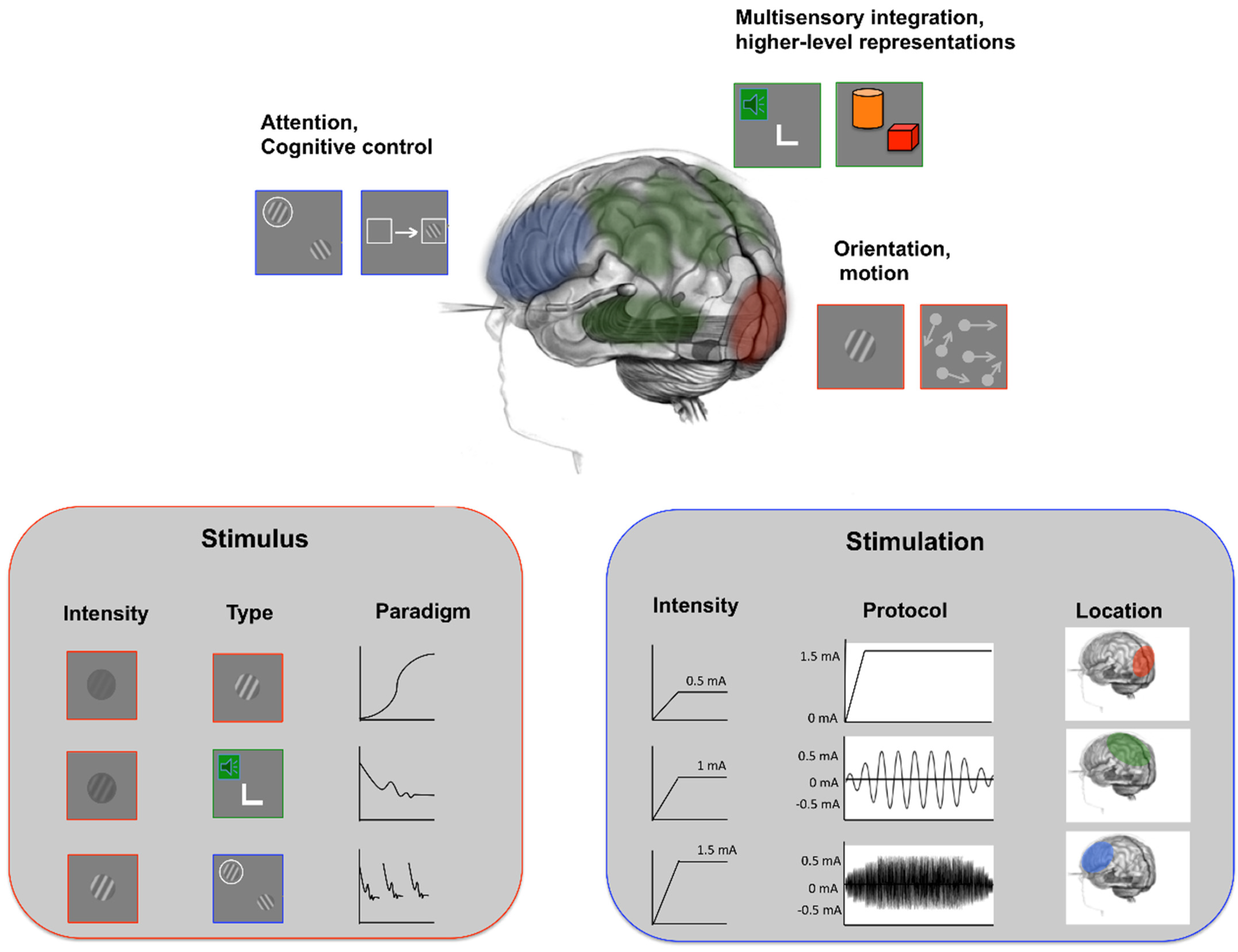A detailed and comprehensive caption for the image described by the three different people would be:

"This is a detailed horizontal rectangular illustration against a white background, depicting an annotated human brain with various regions highlighted in different colors: blue, green, black, gray, and brick red. The brain illustration is central to the image, surrounded by explanatory elements on either side. To the left, there are squares organized under the headings 'Attention' and 'Cognitive Control.' On the right, upper squares are labeled 'Multi-Sensory Integration' and 'Higher Level Representations,' while the lower squares are titled 'Orientation' and 'Motion.' Below these, there are two larger rectangular diagrams with gray backgrounds and rounded corners, displaying various graphs and charts. These rectangles are labeled 'Stimulus' and 'Stimulation,' including detailed columns for 'Intensity Type,' 'Paradigm,' 'Protocol,' and specific brain location associations, illustrating complex neurological data and activities."